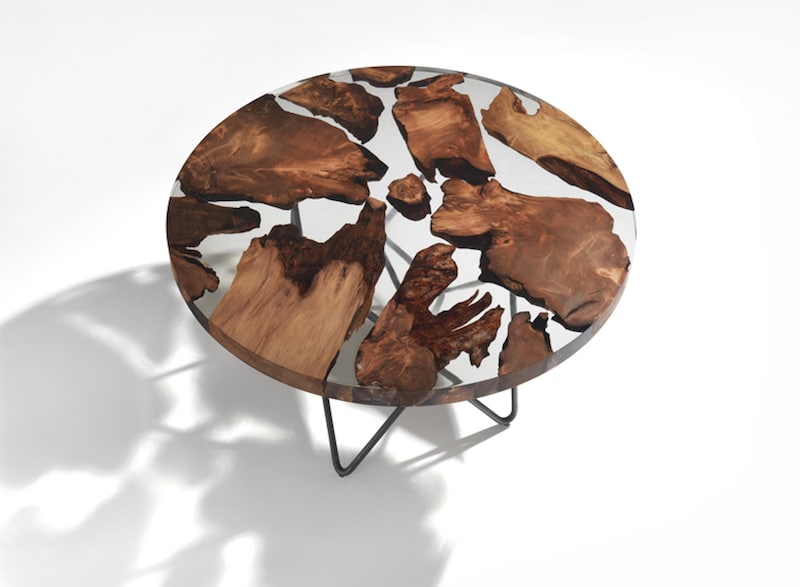This photograph features a round table with a unique design set against a pristine white gradient background. The table, appearing to be a coffee table or perhaps a dining table, has a clear glass or resin surface embedded with various pieces of wood. The woods, displaying a range of light to dark browns, are arranged decoratively in a ring pattern with distinct grainy textures and varied shapes, akin to slabs of meat. Below the tabletop, metal legs or stands support the structure. The glass or resin top showcases intricate details of the wood slices, highlighting different lines, cuts, chips, and textures. The table casts a subtle shadow on the white background, adding depth to the minimalist setting. The table stands approximately five to six inches in height and maintains a clean, straight-edged round form throughout.